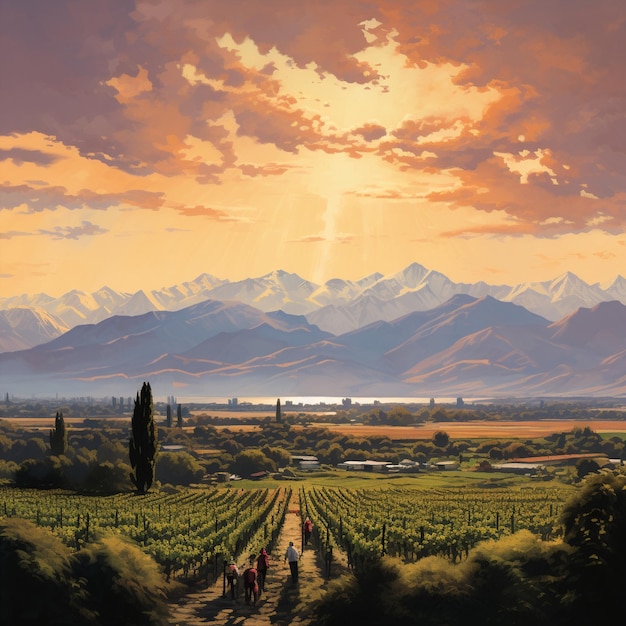This painting showcases an expansive outdoor nature scene dominated by a vibrant vineyard. The foreground is filled with an array of large, green bushes that extend across the entire width of the painting. These bushes vary in shades of green from light to medium. Beyond the bushes lies a vast grape orchard, meticulously planted in rows that stretch from one side of the canvas to the other. Dark wooden posts punctuate the vineyard, supporting the orderly rows of plants. A light brown dirt pathway splits the vineyard, leading into the distance where three figures, possibly tending the vineyard, walk alongside a solitary horse.

The middle ground of the painting reveals several scattered one-story buildings and homes, predominantly white with one prominent brown structure, suggesting a rural settlement or farmhouses. A sprawling dirt field lies beyond these buildings, which meets a dense cluster of trees. Further back, a grand mountain range, with brown hues transitioning to snowy white peaks, spans the horizon. This mountainous backdrop serves as a dramatic contrast to the lush vineyard in the foreground.

The sky above is a striking orange, filled with darker orange and purple clouds. The sun's rays pierce through the clouds, casting a warm glow across the mountaintops and the entire scene below. The light captures the serene yet bustling life of the vineyard, the contrasting colors and textures of the landscape, and the ethereal beauty of the distant mountains.